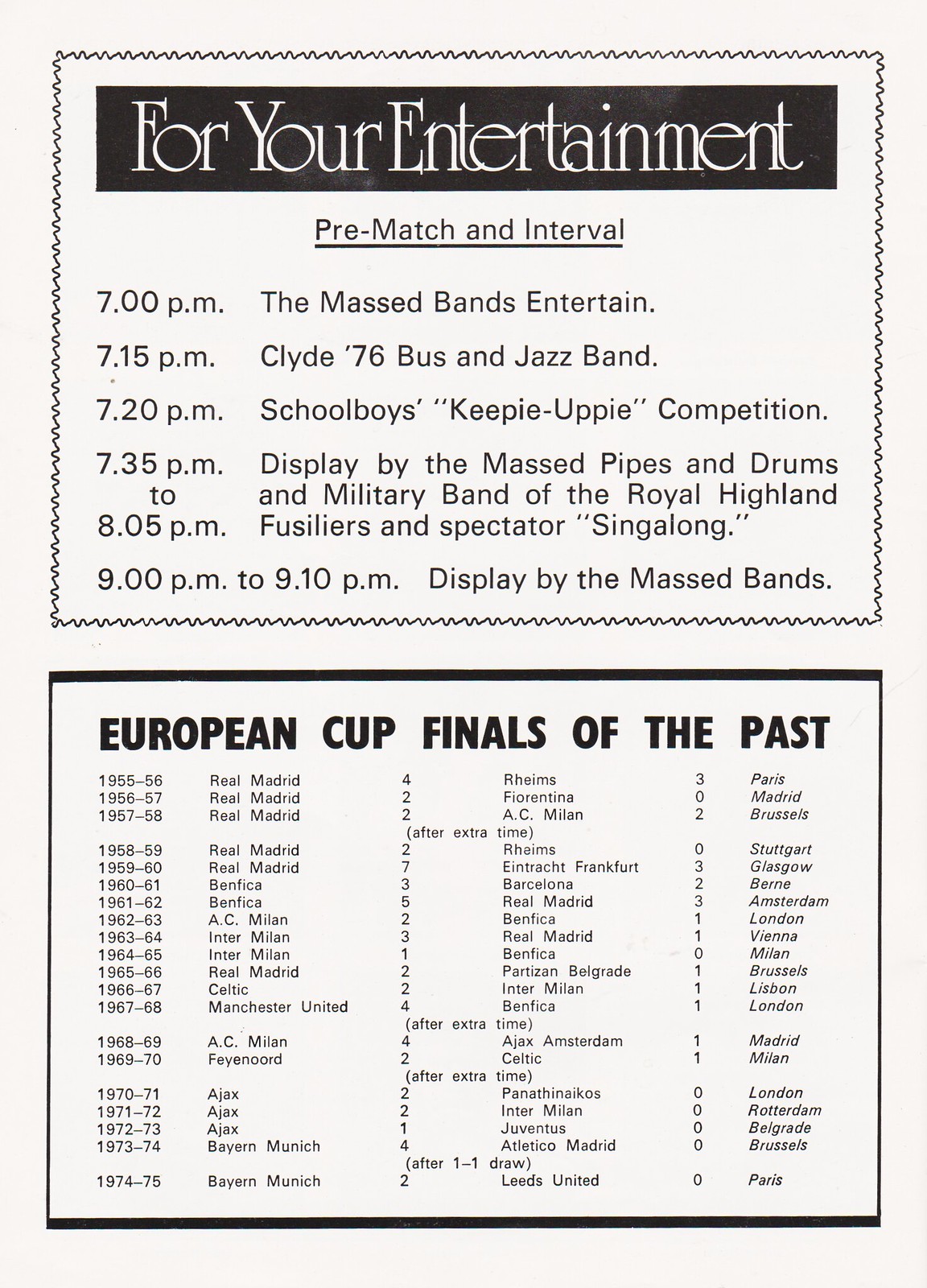The image presents a promotional page for the European Cup Finals of the past, styled in black and white and divided into two equally-sized rectangular sections with borders. The top section features a bold heading in white text against a black background, reading "4-Year Entertainment." Beneath the heading, there's an underlined subheading "Pre-Match and Interval" followed by a scheduled list of entertainment events that run from 7 p.m. to 9 p.m. Starting at 7 p.m., the list includes performances by masked bands, at 7:15 p.m., the Clyde 76 bus and jazz band, at 7:20 p.m., a schoolboys' keepy uppy competition, at 7:35 p.m., a display by the masked pipes and drums along with the military band of the Royal Highland Fusiliers, and ending with a spectator sing-along at 8:05 p.m. The entertainment sessions wrap up with another display by the masked bands from 9 p.m. to 9:10 p.m. The bottom section is titled "European Cup Finals of the Past" in bold black text and provides a chronological list of the European Cup winners, starting from 1955-56 with Real Madrid, followed by the consecutive victories of Real Madrid in 1956-57 and 1957-58. This visually distinct and thoroughly organized promotional page effectively highlights both the historical significance of past European Cup finals and the vibrant pre-match entertainment schedule.